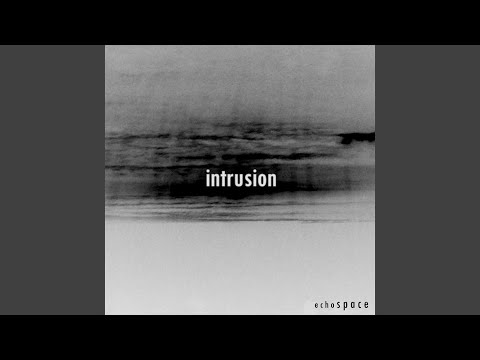This image, reminiscent of an album cover, features a dark gray background with a black strip at the bottom. In the center, a white square contains a blurred black smudge that evokes a sense of rippling water or possibly waves. This smudge is accompanied by shadowy streaks of black and gray extending upward. Central to the white square, in lowercase sans serif font, the word "intrusion" is prominently displayed in white text. At the bottom left corner of this white area, in smaller black lowercase sans serif text, is the name "echo space," with the word "echo" appearing slightly smaller than "space." The overall composition is a horizontal rectangle with a subdued, monochromatic color scheme.